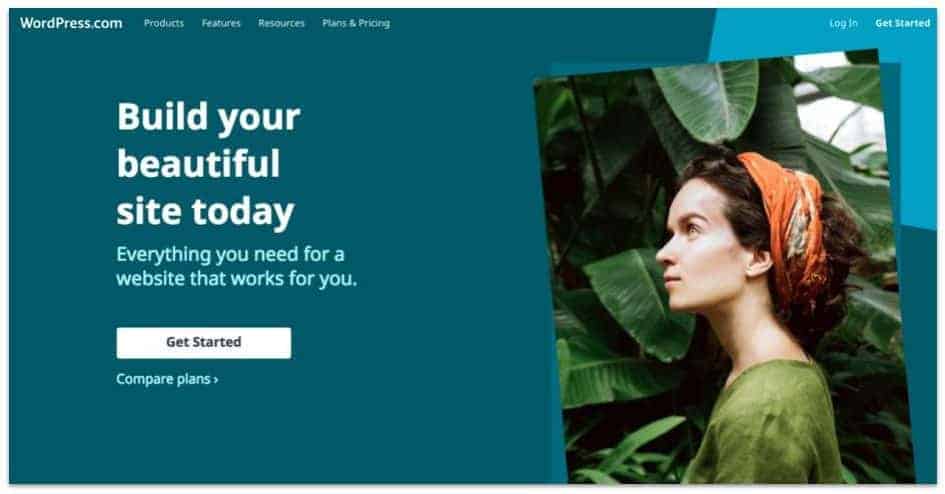This screen grab showcases the homepage of WordPress.com, which features a sleek, teal green-colored banner across the top. The WordPress.com logo is prominently displayed on the left in bold font, while navigation links for "Products," "Features," "Resources," and "Plan & Pricing" are arranged to its right. At the upper right corner, there are two call-to-action buttons: "Log In" and "Get Started."

The main body of the webpage is split evenly. On the left side, there is a textual section with the headline "Build your beautiful site today." Accompanying it is a subheadline that reads, "Everything you need for a website that works for you," followed by a "Get Started" button and a link to "Compare Plans."

On the right side, there's an image of a woman seen from mid-arm up, wearing a green top. She faces left, towards the text, and her brown hair is held back by an orange bandana. She stands in front of a backdrop of large, leafy green plants, adding a natural and earthy element to the composition.